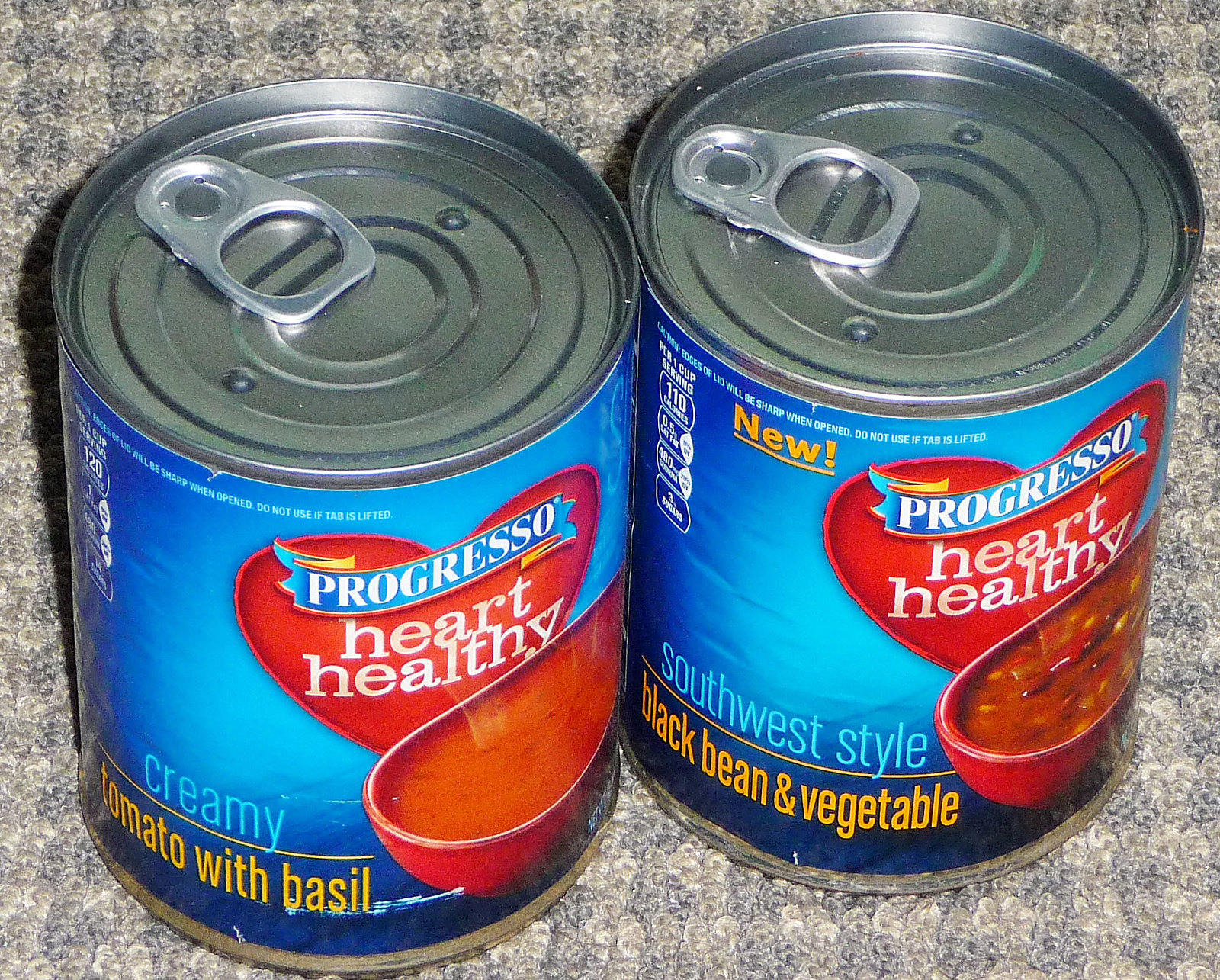This photograph showcases two sealed vacuum cans of Progresso's Heart Healthy soups. The first can is Creamy Tomato with Basil soup, prominently displaying "120 Calories" and "Heart Healthy" on the label, likely indicating the calorie count per serving. The second can, a new flavor of Southwest Style Black Bean and Vegetable Soup, boasts "110 Calories per One Cup Serving" and also features the "Heart Healthy" designation. Both cans are equipped with convenient pop-top lids. The labels, adorned in shades of blue, illustrate the soup varieties: the Creamy Tomato with Basil is depicted with a bowl of tomato soup garnished with small green herbs, and the Southwest Style Black Bean and Vegetable Soup shows a hearty mixture of beans and vegetables. The cans are placed on a grayish, off-white carpeted mat, providing a neutral backdrop.